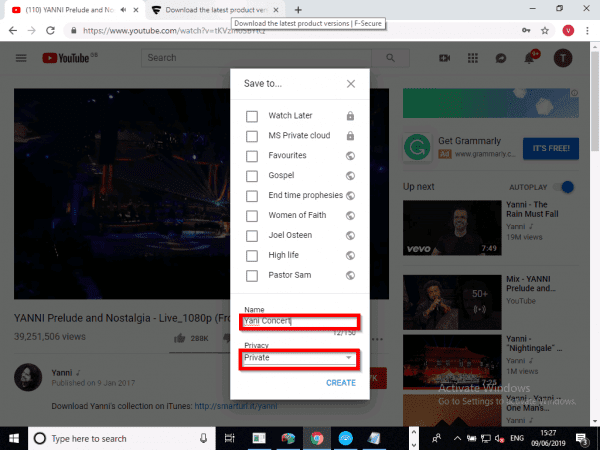This image is a detailed screenshot of a web page. In the upper left corner, there is a browser tab titled "Yanni Prelude," marked by a small red YouTube icon. Adjacent to it on the right is another tab with the title "Download the latest product." Directly beneath these tabs is the address bar displaying "www.youtube.com."

A small white pop-up box overlays the page, featuring gray text. The title at the top of the box reads "Download the latest product versions." Below this title, in the upper right corner of the box, there is a small "X" icon for closing the pop-up.

The pop-up box, which is elongated vertically, presents a menu of save-to options. The options listed from top to bottom are: 
1. "Watch Later"
2. "MS Private Cloud"
3. "Favorites"
4. "Next Gospel"
5. "End Time Prophecies"
6. "Women of Faith"

Each option is clearly delineated, and the overall layout is clean and user-friendly.